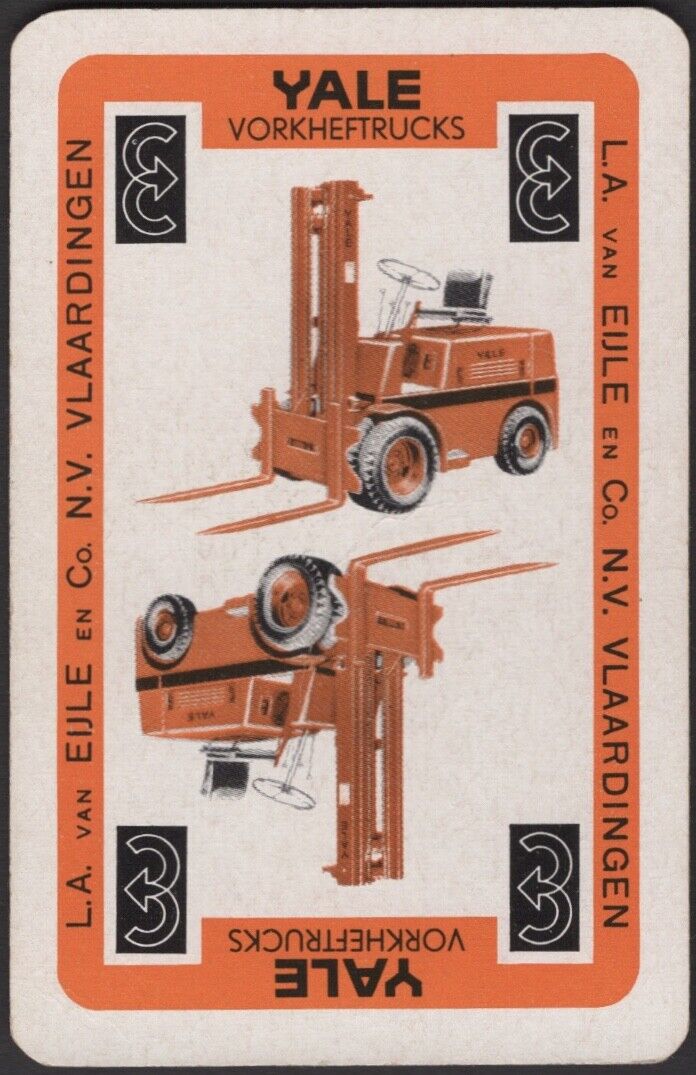This image is a vintage advertisement page featuring an orange border with text reading "Yale Vorkheftrucks" at the top and bottom, and "L.A. Van Elgin Co. N.V. Vlaardingen" written along the sides. The paper has a slightly grayed, aged look. Inside the border, each corner features a black triangle with a white numeral '3' and an arrow. The central portion showcases a detailed drawing of a red forklift truck. The forklift has a black cushioned seat, a steering wheel, and several levers for operation. The top half of the advertisement shows the forklift right side up, while the bottom half mirrors the image upside down, making it reversible.